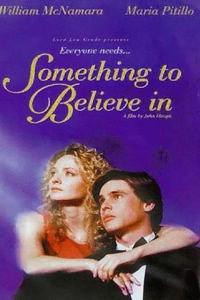The image is a vertically oriented movie poster with a deep blue background, featuring a male-female couple towards the bottom. The woman, with long blonde curly hair and wearing a red dress, has her left arm wrapped around the man's neck, while her right hand clasps her left arm. The man, who has brown hair and is dressed in a black tuxedo jacket with a black bow tie and a white shirt, stands slightly below and to the right of the woman. They both gaze towards the top left corner of the image. At the top of the poster, the names "William McNamara" and "Maria Petillo" are printed in gold text on the left and right corners, respectively. Below these names, in elegant gold script, is the title of the movie, "Something to Believe In," flanked by the phrase "Everyone Needs" in smaller gold text above it. Additionally, there is an indistinct line of text, possibly reading "a film by John Blau," located just below the title. Overall, the sophisticated gold lettering and intense blue background suggest a potentially inspirational or religious theme for the film.